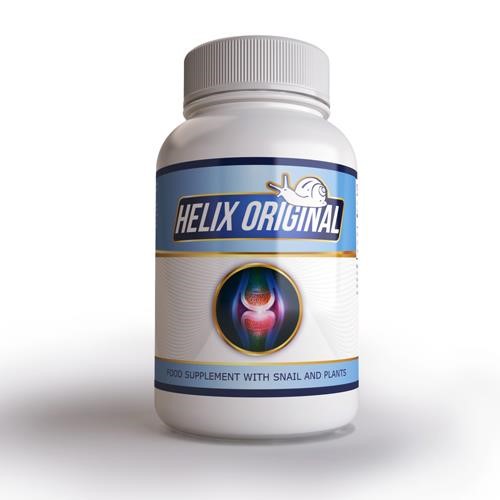This image depicts a white plastic bottle of a joint supplement, likely intended for human consumption. The bottle features a white plastic cap and a detailed label adorned with several key elements. At the top of the label, within a gold-bordered blue rectangle, the brand name "Helix Original," written in all white, capital letters, is prominently displayed alongside a snail logo. Below this section, the central part of the label showcases an illustration of a knee joint, highlighting the bones and a red area indicative of inflammation, all set against a blue background and framed in gold. The label further includes a gold circle with a blue background accentuating the joint imagery.

Further down, the label displays gold and blue stripes with the text "Food Supplement with Snail and Plants" integrated within it. A small section of the label highlights a white area with a blue accent and additional details, including a semi-golden circle. The bottle rests on a flat, white surface, casting a subtle shadow, which enhances the overall presentation. The design incorporates various colors – white, blue, gold, red, orange, yellow, pink, and green – combining to create a visually appealing product package.